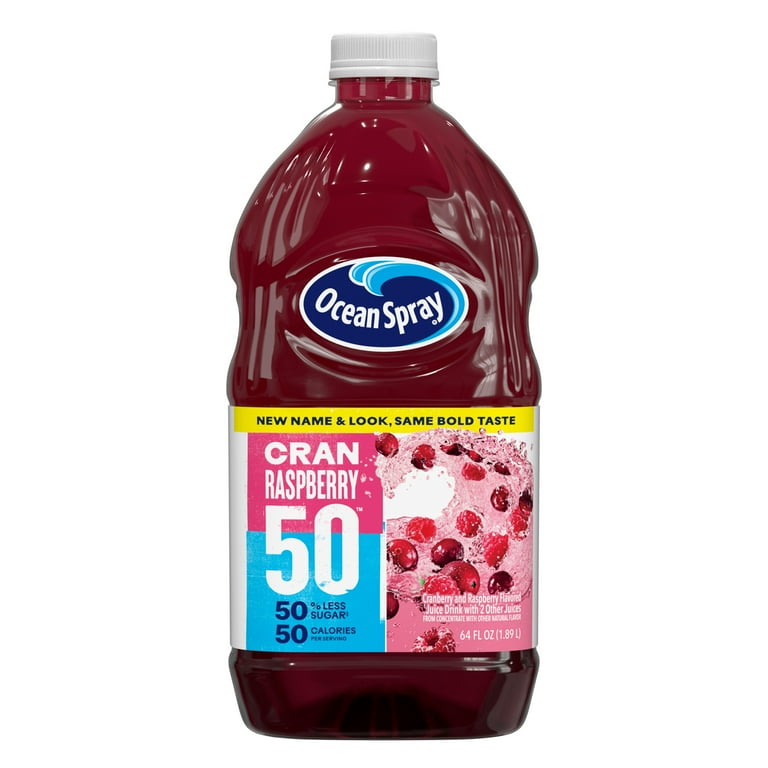This image is a close-up of an Ocean Spray Cranberry Raspberry juice bottle against a white background. The plastic bottle is filled with a dark reddish-pink liquid and has a white screw cap. The Ocean Spray logo, located towards the middle of the bottle, features an oval design in dark blue with "Ocean Spray" in white letters, accompanied by two blue waves on the right side. At the top of the label, a yellow stripe with black text reads, "New Name and Look, Same Bold Taste." The main label, positioned towards the bottom of the bottle, includes a bold "Crayon Raspberry 50" in white text. Surrounding this, additional text in blue notes "50% less sugar" and "50 calories per serving." The label's design also incorporates a vibrant pink wave with images of cranberries and raspberries scattered throughout. The bottle contains 64 fluid ounces (1.89 liters) of juice.